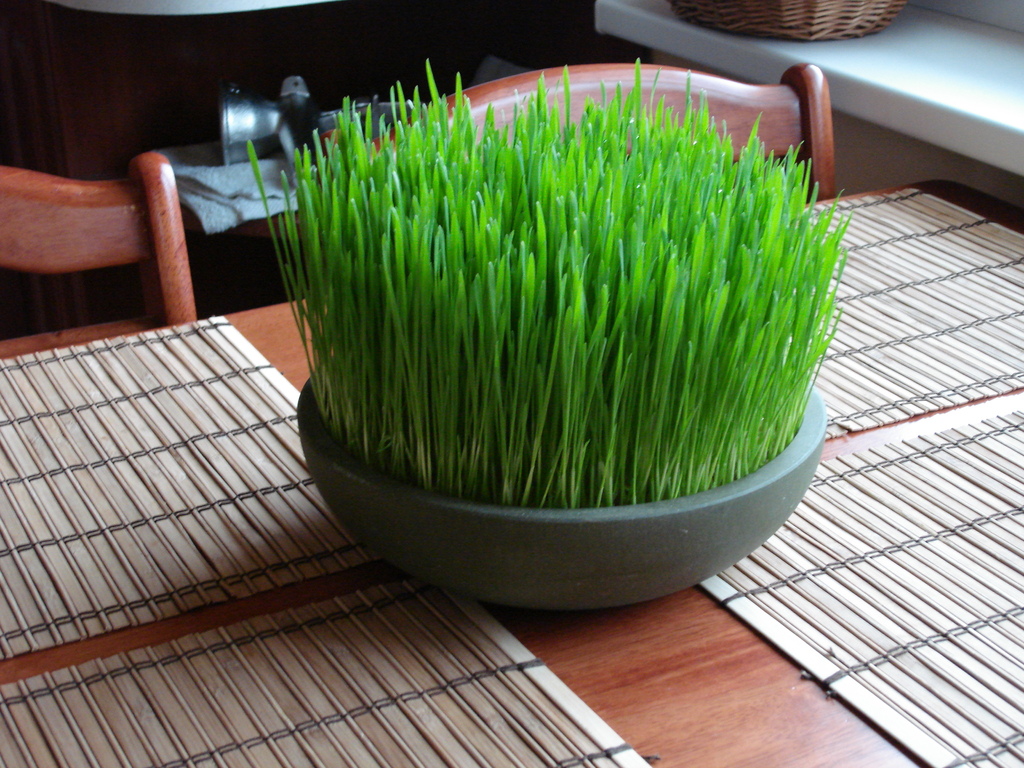In this color photograph, taken at a kitchen table, a dense patch of tall green grass, with light and dark green blades, grows from a round gray stone or ceramic dish at the table's center. The table is a medium brown wood, and surrounding the dish are four silver-colored wire racks that resemble oven racks, each possibly covered by paper or beige slats acting as placemats.

In the upper left-hand corner, part of a matching wooden chair is visible, and another chair's top can be seen behind the grass. The upper right-hand corner reveals a white windowsill, partially obscured by the bottom of a wicker basket, with sunlight casting shiny highlights on the right side of the grass and creating shadows on the left. The background of the room is dark, but hints of a white towel and a bucket suggest a seating area nearby.